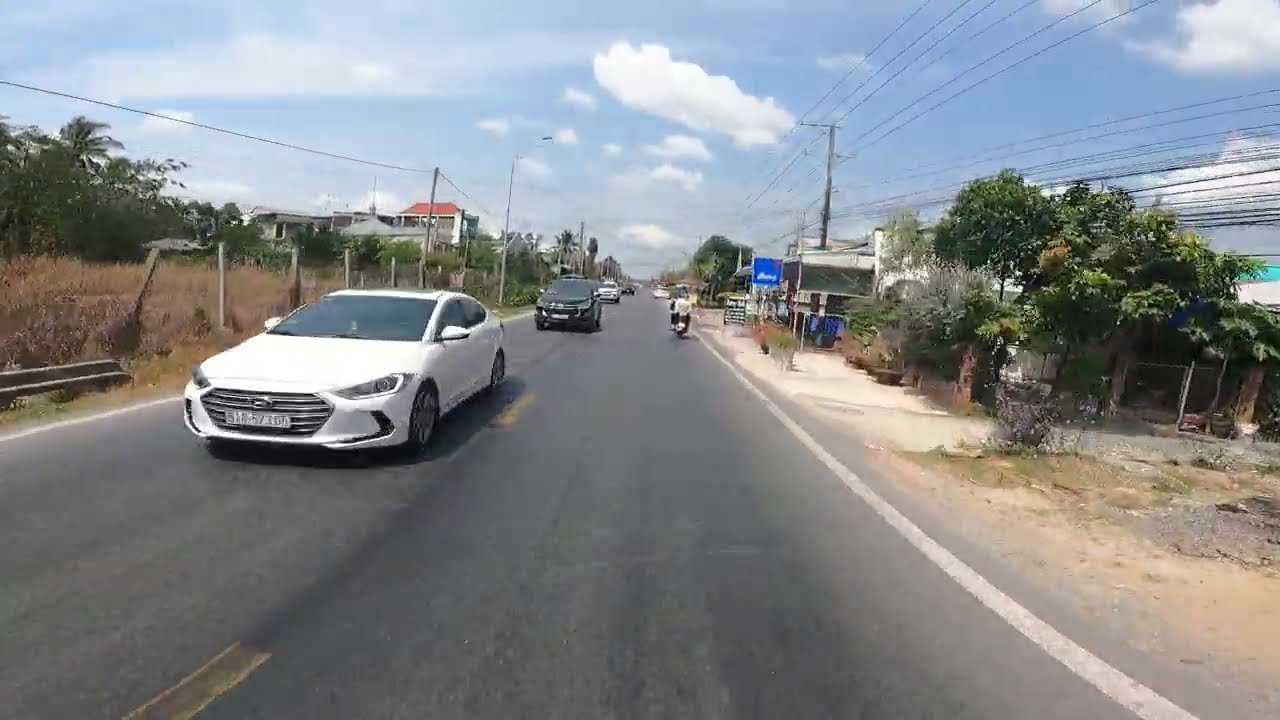The image depicts a rural two-lane asphalt road with clearly marked white edges and a yellow dotted centerline dividing the lanes. The sky is a light blue adorned with white clouds, contributing to a clear and pleasant atmosphere. In the lane of oncoming traffic, three vehicles are visible: a white four-door sedan with a white and black license plate leading, followed by a black SUV, and then a white truck. Heading the opposite direction on the right side is a person riding a moped, dressed in a white shirt and black pants. To the left side of the scene, there's a mix of brown brush and smaller trees, and a more distant building is faintly discernible. On the right side are multiple square buildings with flat roofs, accompanied by businesses and a prominent blue sign, although its text is unreadable. The area appears sparse and dry, suggesting a hot climate possibly reminiscent of regions like India or Pakistan. Features such as telephone poles and wires run alongside both edges of the road, adding to the rural scenery. There is no sidewalk, and a variety of green potted plants are situated near the white buildings, enhancing the overall rural and somewhat arid setting.